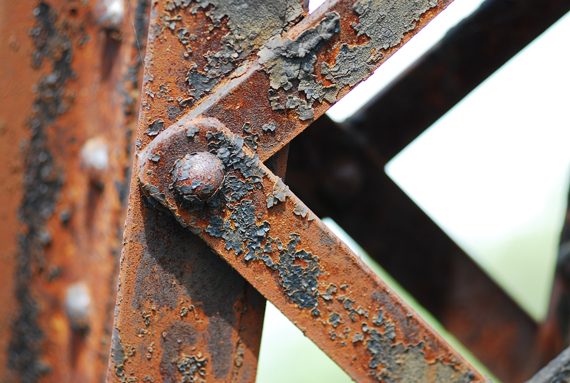This color photograph, in landscape orientation, captures a detailed close-up of an aging and heavily rusted metal structure. The primary focus is on a vertical beam on the left, painted in a chipping dark gray that has oxidized over time, revealing a mix of rusted brown and brick-red tones. This beam features three silver-toned metal studs arranged in a vertical row. From the top and bottom right of the image, two thinner rusted and decayed metal brackets extend, meeting at a central, rounded bolt that secures them together. The backdrop, a blurred white surface with hints of sunlight, suggests an outdoor setting, further emphasizing the prolonged exposure to the elements that has led to the metal's extensive weathering. Alongside the main structure, additional rivets and bolts can be seen, slightly shadowed and similarly corroded, contributing to the intricate texture and narrative of aged metalwork portrayed in the photograph.